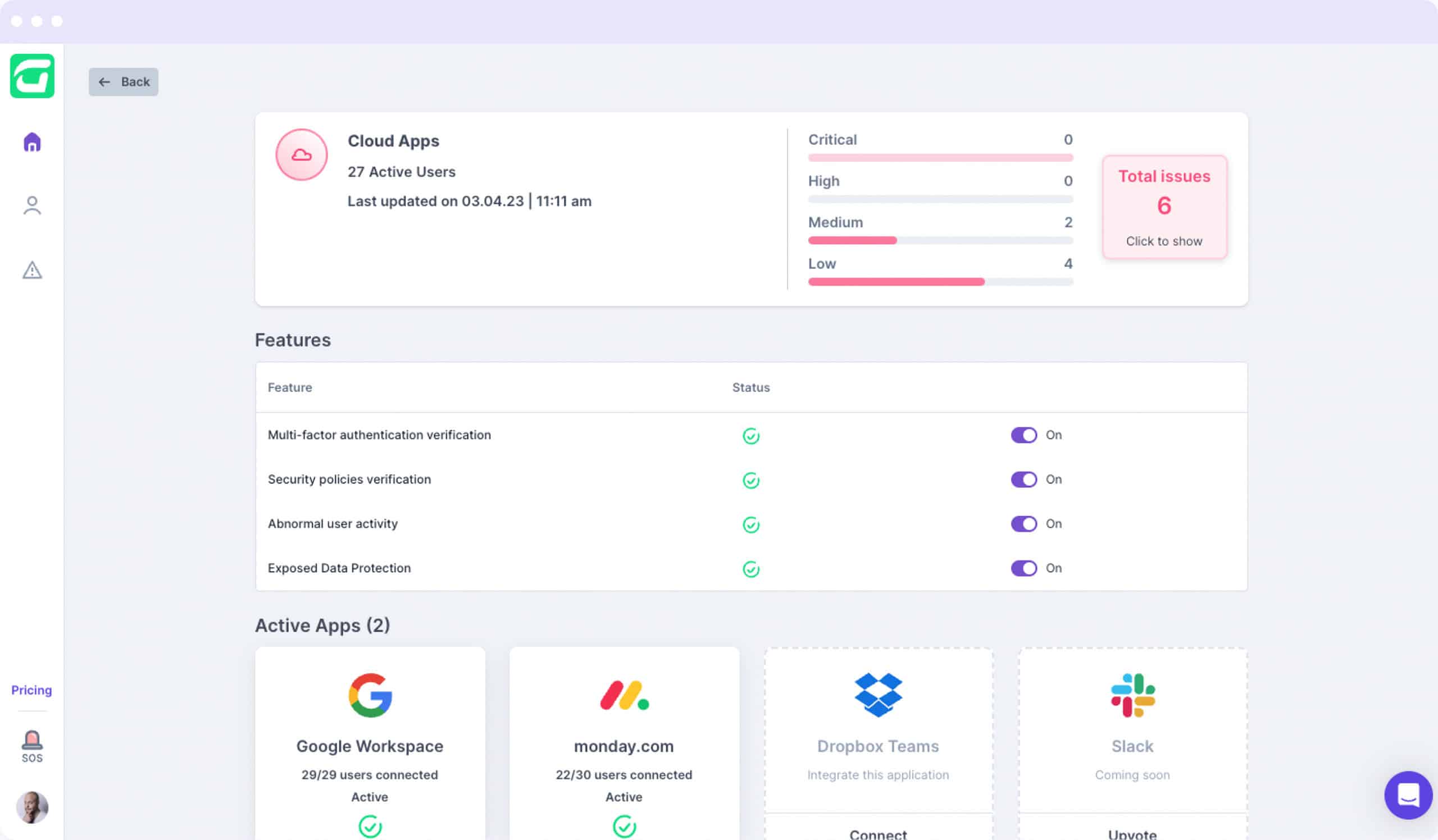This screenshot captures a settings page on a website, characterized by a lavender header featuring three white dots arranged horizontally in the top left corner. Below the header, a white sidebar prominently displays various icons and text elements. The sidebar begins with a green, rounded square containing a white, abstract 'G'. Beneath this are three icons: a purple house, a gray person, and a gray triangle with a gray exclamation point.

Towards the bottom of the sidebar, the word "Pricing" is written in purple text, followed by a thin gray line. Below this, an orange warning light icon is present, accompanied by the gray text "SOS". At the very bottom is a circular profile picture of a man.

To the right of the sidebar lies the main body of the page, set against a light gray background. At the top left of this area is a medium gray rectangle with rounded corners featuring medium gray text and a left-pointing arrow labeled “Back.” Directly below and to the right is a white rectangle. Inside, a pink gradient circle with a dark pink cloud icon occupies the top left. Adjacent to this, gray text reads "Cloud Apps, 27 active users, last updated on 03.04.23, 11:11 am."

Separated by a vertical gray line, the right portion of the white rectangle hosts a series of four colored bars. The first bar, labeled "critical," is pink. The second bar, labeled "high," is light gray with zero indication. The third bar is a combination of dark pink and light gray, labeled "medium," filled about one-third with dark pink. The final bar, labeled "low," is filled to about two-thirds with the same colors, representing four instances.